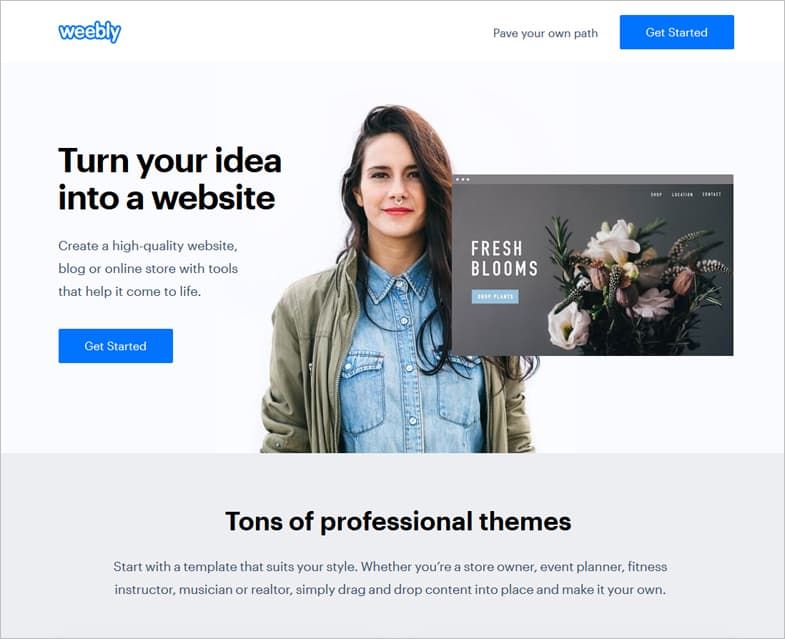The desktop screenshot features the Weebly homepage. At the top left, the word "Weebly" is prominently displayed in a clean, sans-serif font. The background is predominantly white with light gray accents and a darker gray at the bottom. To the right of "Weebly," a motivational tagline reads, "Pave your own path." Adjacent to this, a blue button says "Get Started."

In the central area of the page, a headline proclaims, "Turn your idea into a website," accompanied by an image of a beautiful young woman. She has Caucasian skin, auburn (possibly brunette) hair, a nose ring, and a faint smile. She is dressed in a collared denim shirt layered with a light green sweater.

Below the headline, additional text in bold black font explains, "Create a high quality website, blog, or online store with tools that help it come to life." Another blue "Get Started" button is situated underneath this text.

To the right of the woman, there is a screenshot of a Safari browser showing a website titled "Fresh Blooms," which appears to be an online shop for plants. The image showcases a variety of flowers.

In the bottom section with a darker gray background, bold black text highlights, "Tons of professional themes." It elaborates, "You can start with a template that suits your style, whether you're a store owner, an event planner, a fitness instructor, a musician, or a realtor. Simply drag and drop content into place and make it your own."